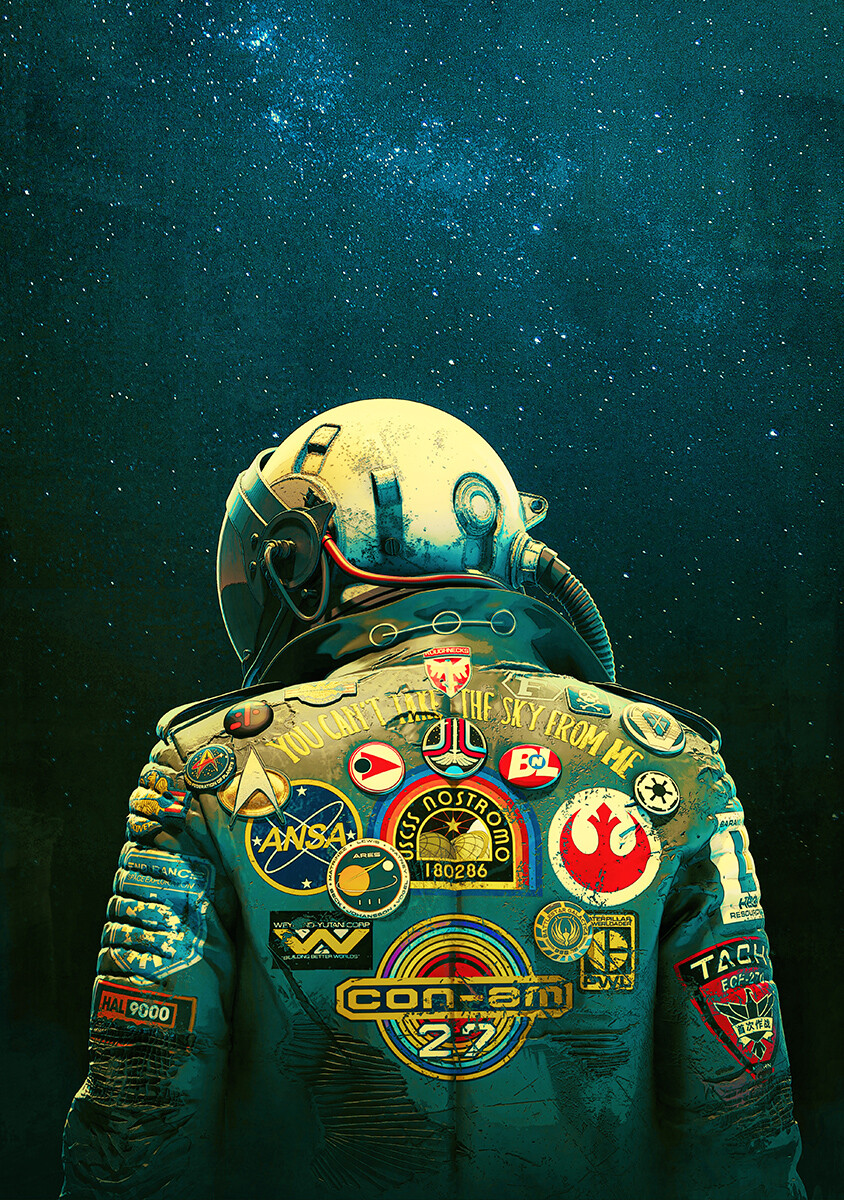The image is a detailed, surreal graphic painting of the back of an astronaut, set against a predominantly black background with swirling blue areas and scattered, varying-intensity white dots symbolizing stars. The astronaut's head, slightly turned to reveal part of the clear visor shield, is covered by an all-white helmet connected by a black hose to an unseen oxygen tank. He wears a black leather jacket adorned with numerous badges and buttons from popular Hollywood movies, including logos from "Star Wars," "Star Trek," "Aliens," and "The Last Starfighter." Prominently displayed at the top of the jacket are yellow text reading, "You can't take the sky from me." The scene evokes the vastness and mystery of outer space, enhanced by the eclectic mix of space-themed memorabilia decorating the astronaut's attire.